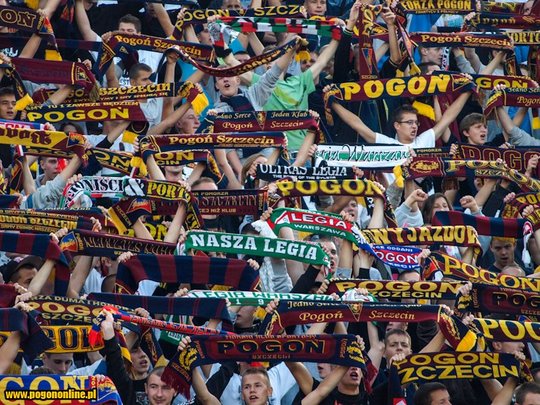The image depicts a large, vibrant crowd of people, seemingly gathered for a protest or a rally. Among the crowd are both men and women, predominantly young men, all holding up colorful banners and signs. The banners display text in a language other than English, with several prominently featuring the words "POGON" and "NASZALASIA." The signs come in various color combinations, including green with white letters, green with red and white letters, navy blue with red and white letters, and yellow letters against a lavender background. The crowd appears energetic and unified, many with their arms raised high, displaying a sense of camaraderie and common purpose. The image conveys a sense of movement and solidarity among the participants, who are dressed in contemporary clothing, making it clear that this is a recent, dynamic event captured in full color.